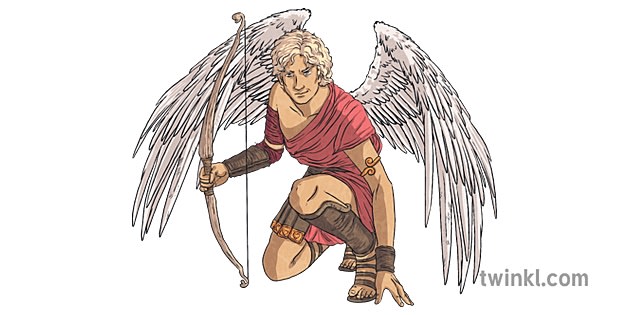This detailed hand-drawn illustration titled "twinkle.com" depicts an angelic figure. The character, a winged blonde man with an ethereal presence, is captured in a crouched position, taking a knee. Adorned in an off-the-shoulder red toga-like top that extends into a leather skirt, reminiscent of a Roman soldier's attire, the angel combines divine and martial elements. He is outfitted with brown, tight leather leggings from the knee down, matched with leather armbands and shin guards. His footwear consists of classic leather sandals. Notably, he brandishes a bow in his right hand, adding to his celestial warrior image. The man has two large, majestic white wings and white hair. A golden arm bracelet adorns his left bicep. The image, set against a stark white background, features the website "twinkle.com" in gray at the bottom right corner.